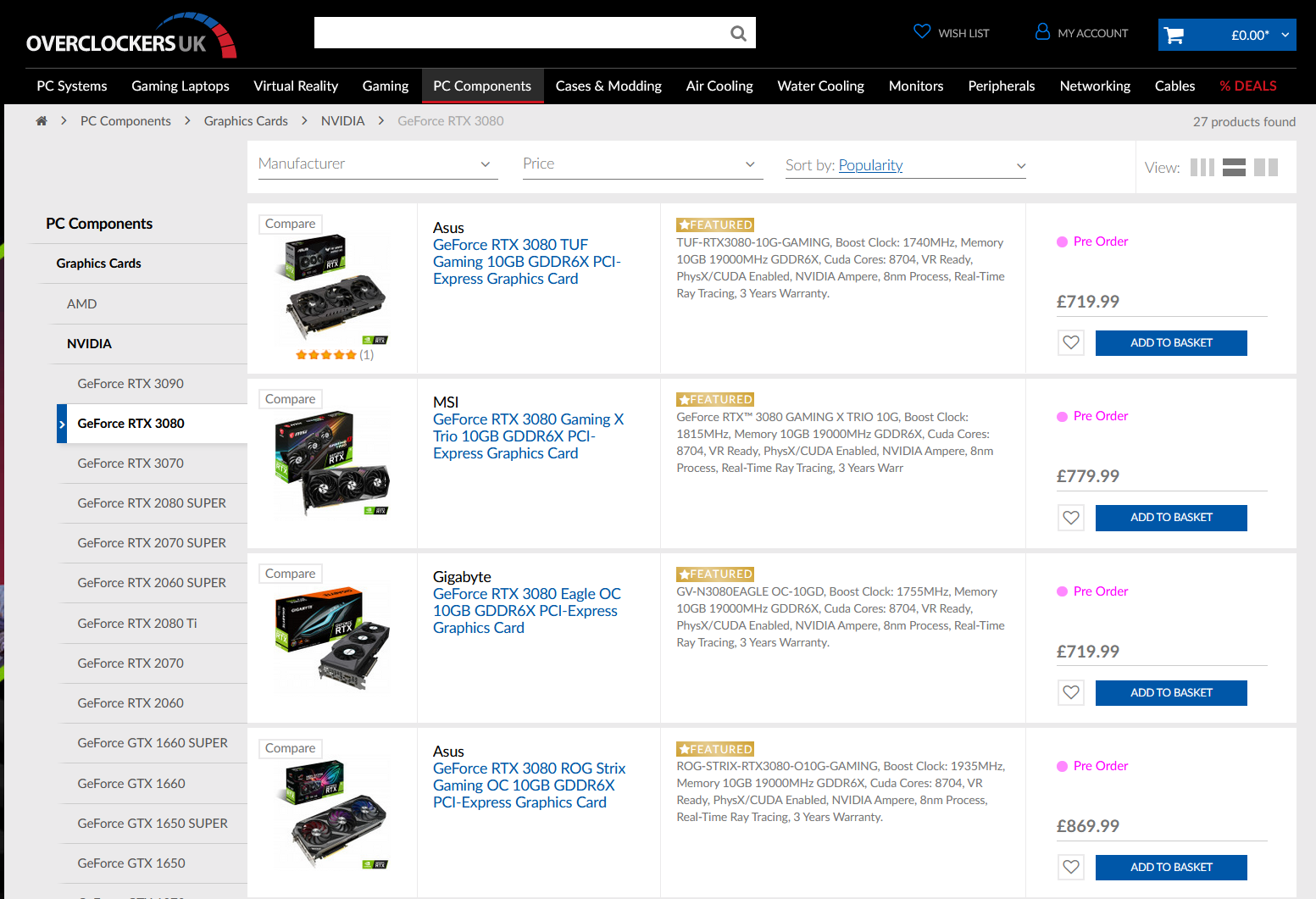The screenshot depicts the Overclockers UK e-commerce website, which specializes in selling computer parts. The header of the site is black, featuring the Overclockers UK logo in white, gray, blue, and red. The site employs blue accent text and occasional red elements for emphasis. 

Prominently placed in the header are a search bar and buttons for accessing the wishlist and "My Account" sections. A dropdown button displaying the cart total is also present, which currently indicates a total of zero pounds, meaning no items have been added to the cart yet.

The top menu features a wide array of categories, including PC Systems, Gaming Laptops, Virtual Reality Gaming, PC Components, Case and Modding, Air Cooling, Water Cooling, Monitors, Peripherals, Networking, Cables, and "Percentage Deals," distinguished in red and preceded by a percentage symbol.

The screenshot specifically highlights the "PC Components" section, with a focus on Graphics Cards. Currently, it displays Nvidia GeForce RTX 3080 models. On the left side, there is a list of different GeForce graphics card models, while the right side presents a series of tables organized into different columns and rows. These tables contain product names, brief descriptions, product photos, and prices, along with options to add items to a wishlist or directly to the shopping basket.